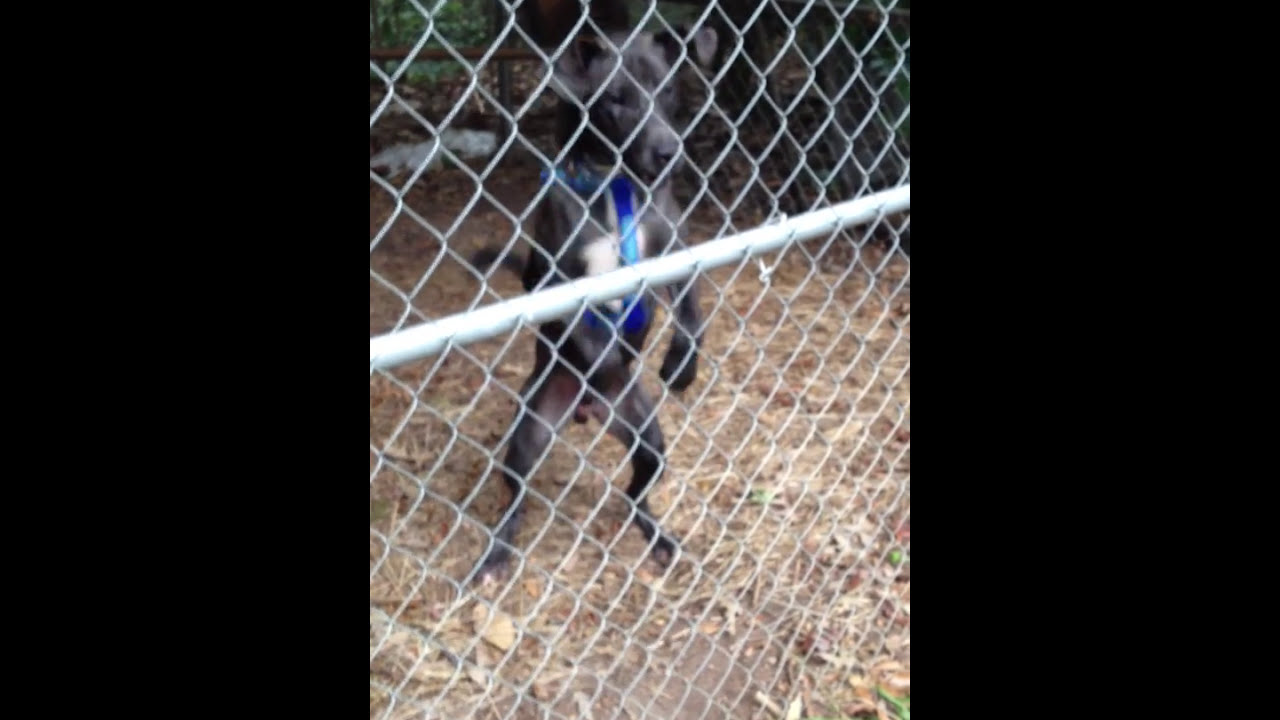In this daytime image, a black dog with drooping ears and a white chest spot stands on its hind legs behind a chain-link fence. The fence features a gray metal bar running through its center. The dog appears to be wearing a blue harness. The kennel floor is scattered with hay and dried leaves, revealing packed brown dirt in bare spots. Black rectangles occupy the sides of the image, creating a framing effect. In the background, a green bush or tree and a brown railing are visible through the fence.